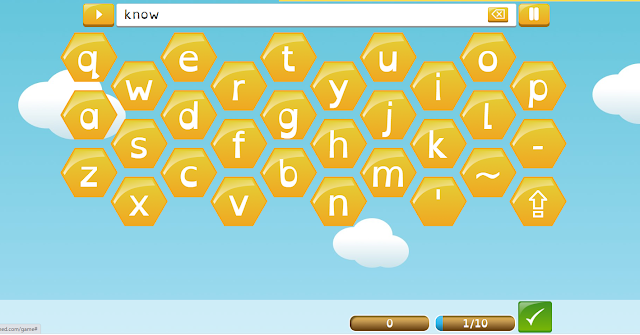A detailed and cleaned-up descriptive caption for the image could be:

"Screenshot of a computer screen displaying a digital drawing rather than a photograph. The background features a blue sky with scattered, puffy white clouds. In the foreground, there's a unique floating QWERTY keyboard; each key is hexagonal and arranged in a hexagonal close-packed grid. Despite the unconventional arrangement, the keys maintain the standard typewriter layout when traced in a zigzag pattern. At the top of the image is a text box with accompanying buttons: an arrow, a backspace, and a pause button. The text box contains the word 'KNOW,' presumably typed using this novel keyboard. At the bottom of the screen, a lighter blue bar stretches across, with some illegible small text in the lower left-hand corner. To the right side of this bar, there are two rounded rectangles: one is brown with the numeral '0,' and the other is brown with a touch of blue, displaying '1/10,' suggesting a progress metric. Further to the right, a green box with a check mark indicates completion or confirmation of some action."